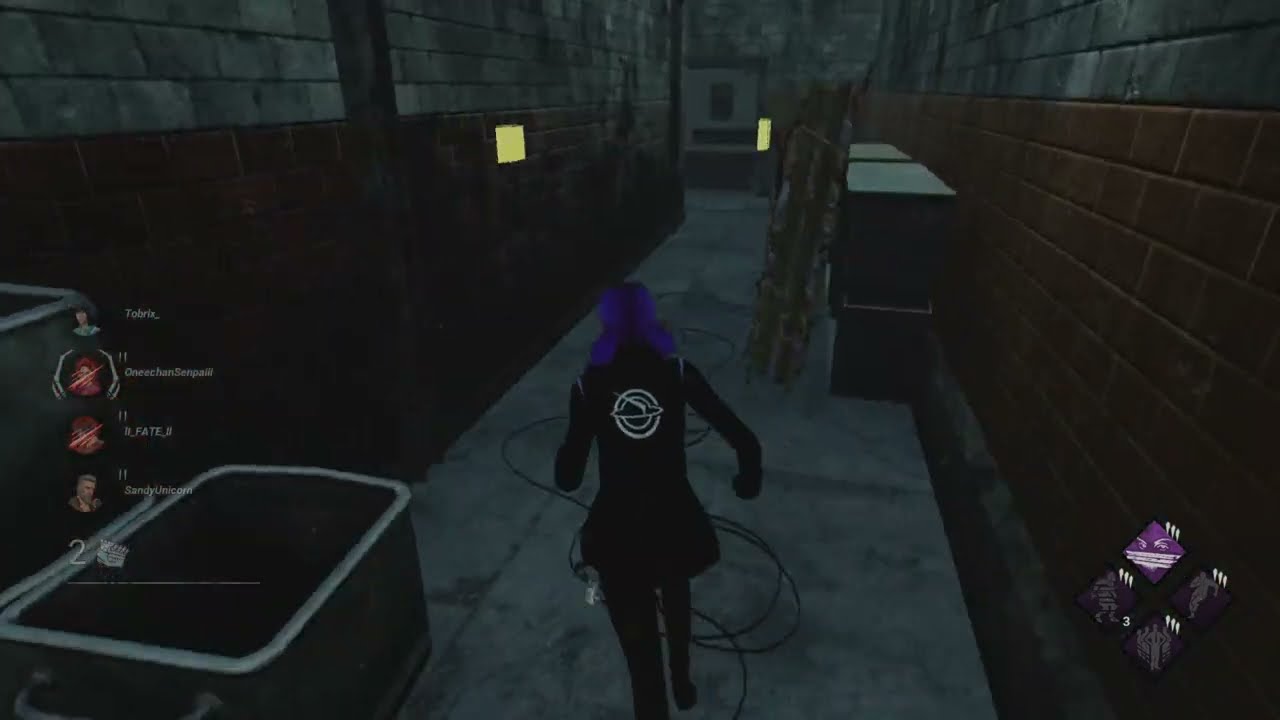The image appears to be a highly detailed, professional still from a video game. The scene captures a dark, ominous alleyway or hallway at night, framed by reddish-brown and gray brick walls on each side. In the foreground, we see the back of a character, possibly a woman, with vibrant purple hair. She is wearing black pants and a black jacket featuring a white spaceship logo on the back. The character appears to be either running or walking purposefully towards a door in the background, suggesting a sense of urgency or pursuit.

The environment is textured with various items: in front of the character, there are ropes or wires, and further along, there might be boxes or stands. The colors in the scene include a pronounced palette of black, white, gray, red, brown, with occasional hints of yellow, green, and a significant dominance of various neutral shades.

Additional game interface elements are visible: in the bottom right corner, purplish squares display different poses the character might adopt. On the left side, there are small player pictures and names arranged in order, likely representing player rankings or statuses. Overall, the image conveys a dark, tension-filled atmosphere, emphasizing the character's mid-action posture within the gritty, urban setting.